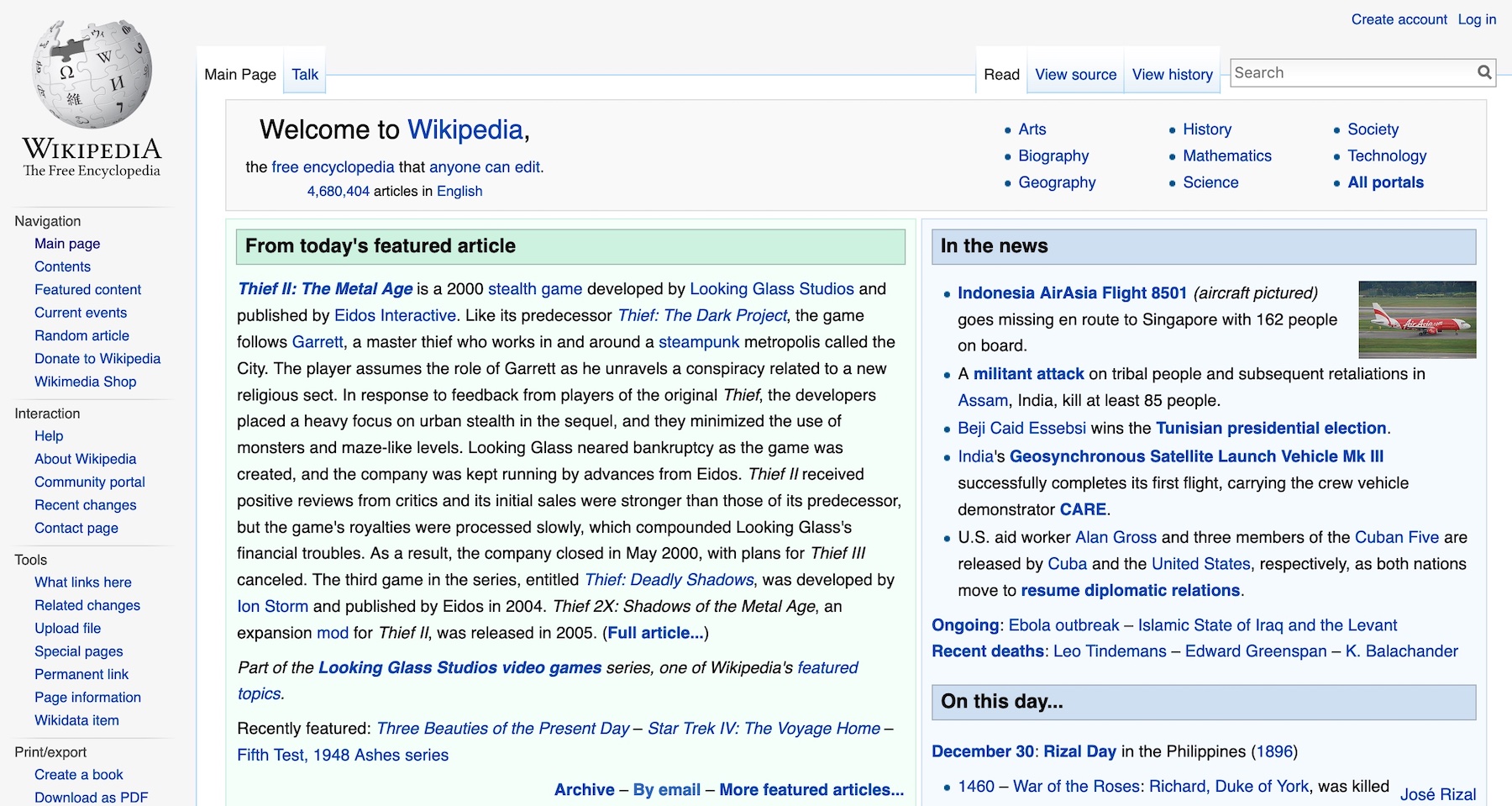The screenshot is of the Wikipedia homepage, displaying a comprehensive overview of the site's vast content and various navigational tools. On the left, beneath the iconic global logo composed of puzzle pieces with the inscription "Wikipedia, the free encyclopedia," a vertical menu presents a multitude of options. These include navigation links such as Main Page, Featured Content, Current Events, Random Article, Donate, and the Wikimedia Shop. Interaction options are also provided, featuring links to Help, About Wikipedia, Community Portal, Recent Changes, and Contact information. Additionally, tools like What Links Here, Related Changes, Upload File, Special Pages, Permanent Link, Page Information, and Wikidata Item are available, alongside print and export functionalities for creating a book or downloading content as a PDF.

The central section welcomes the user to Wikipedia, highlighting major categories such as Arts, Biography, History, Mathematics, Science, Society, Technology, and All Portals. Below this, "Today's Featured Article" is showcased, featuring Thief 2: The Metal Age, a 2000-tech stealth game developed by Looking Glass Studios, accompanied by a brief explanatory paragraph.

To the right, under a teal-colored header, is the "In the News" section, marked by a blue header. It lists current events, including the disappearance of Indonesia Air Asia Flight 8501 and a militant attack in India. Further down, there are additional news stories. Adjacent to this is the "On This Day" panel, listing significant historical events for December 30th, such as Rizal Day in the Philippines (1896) and the death of Richard, Duke of York, in the War of the Roses (1460).

This detailed layout on the Wikipedia homepage provides users with easy access to a wide array of information and interactive options.